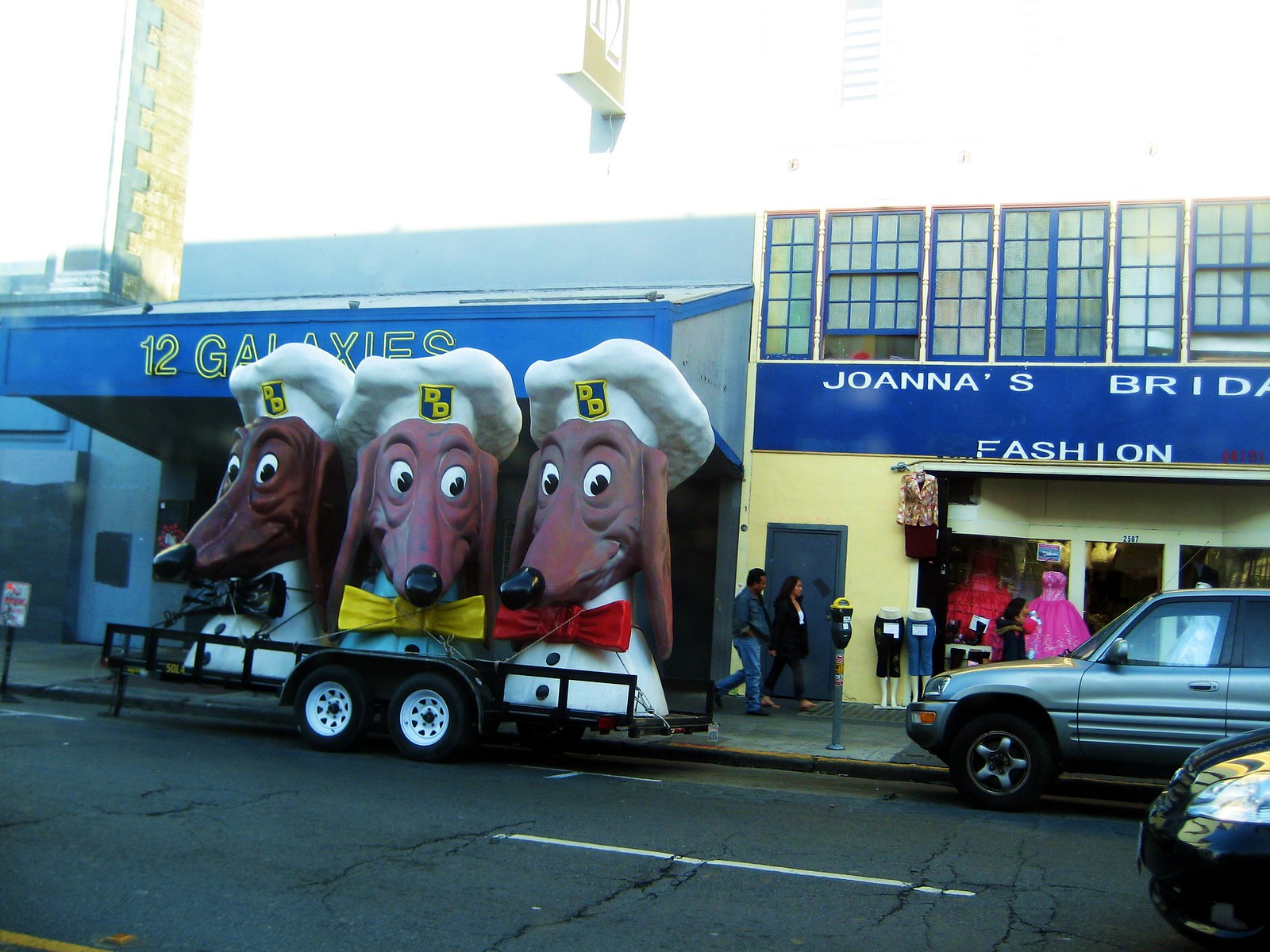The photograph showcases a street scene featuring two distinct stores, "Joanna's Bridal Fashion" adorned with a blue banner and a yellow storefront, and "12 Galaxies" marked with a blue awning and neon signage. In front of the 12 Galaxies store sits a large black trailer displaying three oversized, cartoonish heads resembling Goofy or wiener dogs. Each head is reddish-brown with black noses, long ears, and big white eyes. They wear white chef caps embellished with a blue and yellow crest and are dressed in white shirts with black buttons. The first head dons a black bow tie, the middle a yellow one, and the rightmost a red bow tie. The scene includes an asphalt road with a pale blue car, possibly a CRV, parked in front of Joanna's Bridal Fashion, and two pedestrians walking by the storefronts.